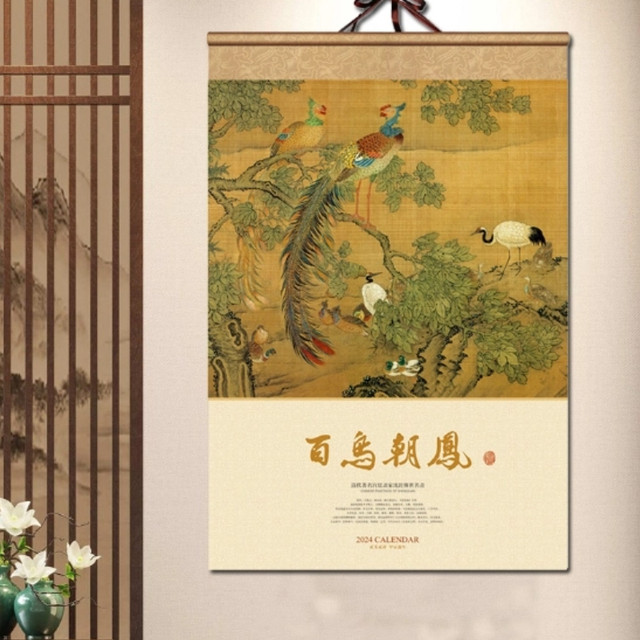The photograph captures a square indoor scene featuring a decorative and detailed wall hanging. Dominating the right side of the composition, a scroll-like calendar is suspended by a brown ribbon. The top portion of this calendar is crafted from thick, gold-toned brown fabric, while the rest is reminiscent of plain paper. The artwork on the scroll depicts a rich, wilderness scene. A prominent brown tree, adorned with green leaves, supports various colorful birds including a peacock and parrots, positioned amidst branches. Additionally, black and white birds such as herons or cranes are visible along the lower right side of the painting. 

Below the intricate bird illustration lies some Asian lettering against a white background, followed by a 2024 calendar printed in black and larger red text. The backdrop of the image reveals a brown-painted wall resembling a mountain landscape, partially obscured by vertical and horizontal wooden slats.

In the lower left corner of the photograph, two green vases with white flowers add a touch of elegance. The overall decorative style leans towards muted, neutral tones, providing a minimalist yet charming aesthetic.